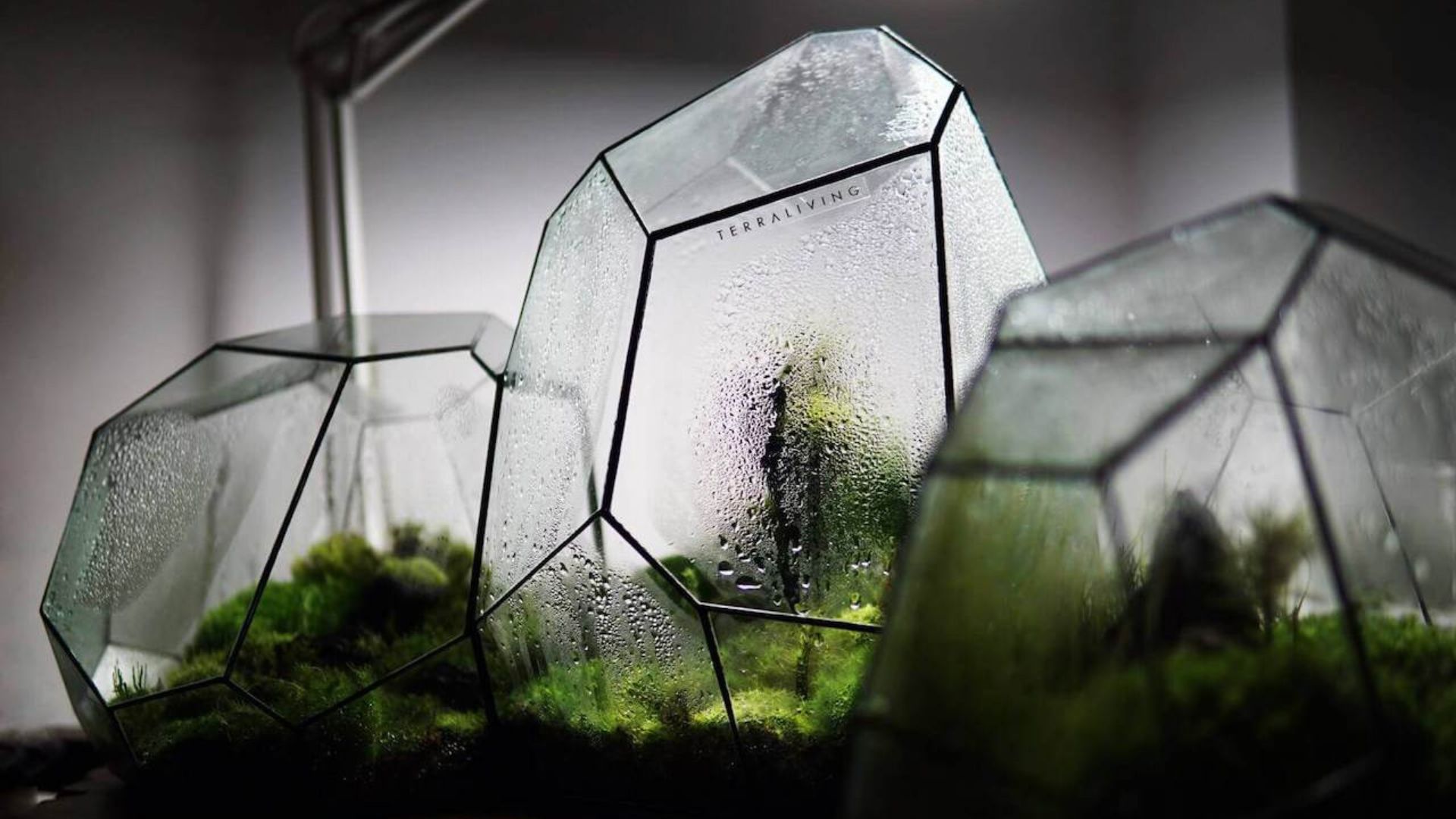The image showcases three uniquely shaped terrariums, each designed with faceted, crystal-like glass panels resembling gemstones. The geometric containers—one tall central piece flanked by two shorter ones—feature multiple hexagonal and octagonal faces that create a gem-like dimension. Inside the terrariums, various plants, predominantly different types of moss, thrive in a miniature garden landscape. The glass surfaces are densely misted with condensation, presenting a foggy appearance that obscures the finer details but hints at the lush greenery within. The middle terrarium bears a label with the text "There are leaving" in black font. Set against a backdrop of artificial indoor lighting, the terrariums are backlit, enhancing their visual appeal. The dim lighting and enclosed setting suggest these terrariums might be part of a display in a museum or a botanical exhibit.